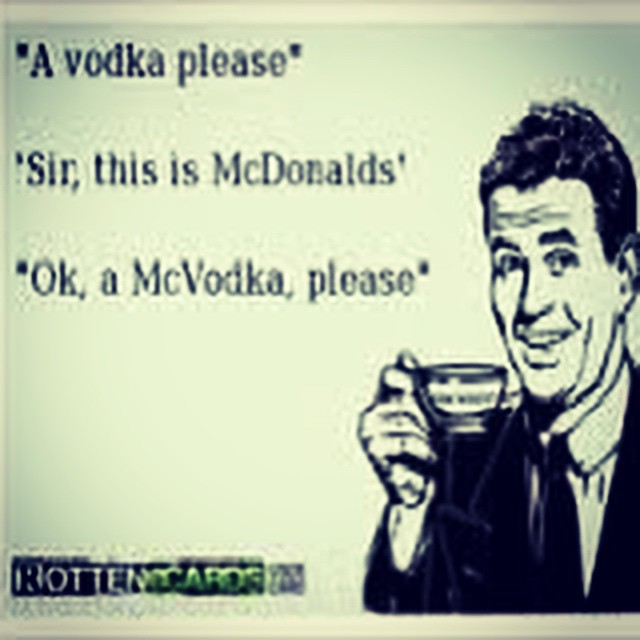The image is a cartoon-style advertisement with a light-colored center that fades into a muted teal at the top and bottom. It is grainy and pixelated, giving it a low-resolution, older meme-style appearance. Positioned on the right side is a black-and-white drawing of a man wearing a suit with a collared shirt and tie. The man, who has short, curly hair and raised eyebrows with wrinkles on his forehead, is holding up a small cup close to his face. He is grinning with his teeth exposed. To the left of the man, there is a humorous dialogue in black text that says, “A vodka please.” Below it, another line reads, “Sir, this is McDonald's.” Following that, the text continues, “Okay, a McVodka please.” The bottom left of the image features the stamp "rotten cards," likely indicating the source of the cartoon.